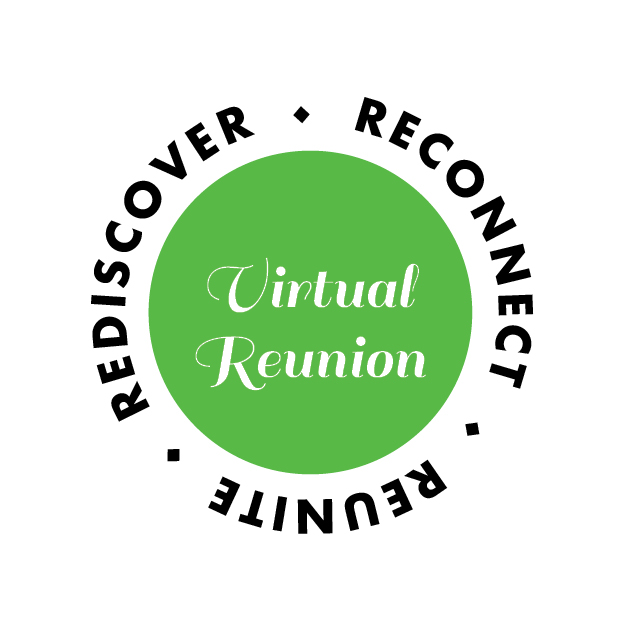On a white background, the central focus is a green solid circle featuring the elegantly scripted text "Virtual Reunion" with an initial capital “V” and “R” and the rest of the letters in lowercase. Surrounding this green circle is a circular pattern of bold black text in all caps that reads "REDISCOVER," "RECONNECT," and "REUNITE." Each word is separated by diamond-shaped symbols, giving a dynamic visual rhythm to the design. The green circle's graceful font contrasts against the bold, straightforward Arial-like font of the surrounding text, blending elegance with clarity.